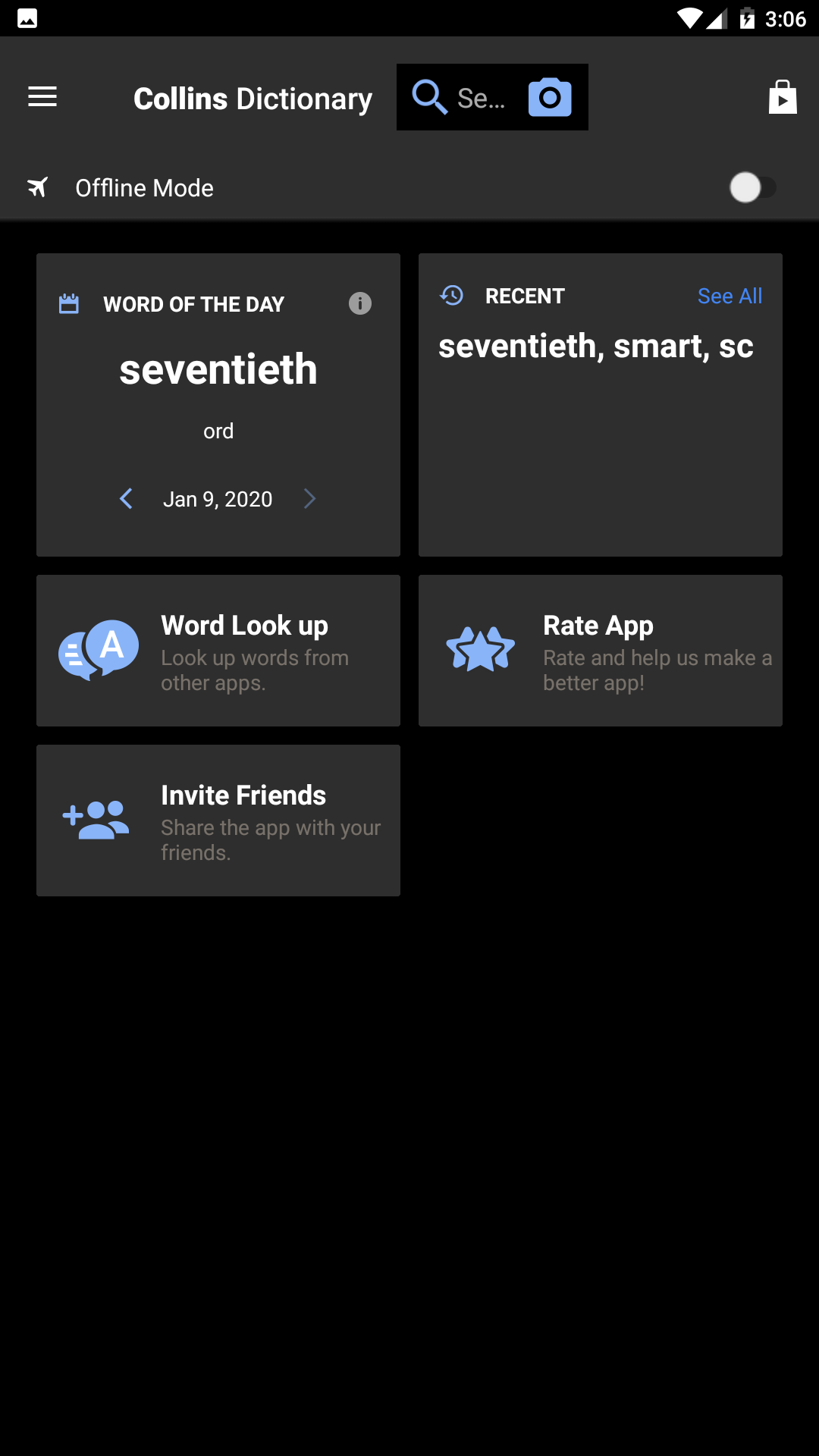Screenshot of a mobile phone interface in dark mode displaying the Collins Dictionary app. The top section of the screen features a black background with various icons: the gallery icon in the upper left corner, and in the upper right corner, icons indicating the Wi-Fi signal, mobile signal strength, battery level, and the current time (3:06). Directly below, there is a gray bar with white text that reads "Collins Dictionary." To the right of this text, there is a black rectangle containing a blue magnifying glass icon, signifying a search field. Further to the left of the search bar, three horizontal white lines are displayed vertically, and on the far right side is a shopping bag icon.

In the lower left corner of the screen, an airplane icon is present with the label "offline mode," accompanied by a toggle switch in the lower right corner that is currently toggled off.

Below this section, on the left side, there is a gray box displaying "Word of the Day: 70th January 9th, 2020," while on the right side, another gray box shows "Recent: 70th smart SC". 

Further down, there are two additional gray boxes. The one on the left reads "Word Lookup: Look up words from other apps," and the one on the right reads "Rate App."